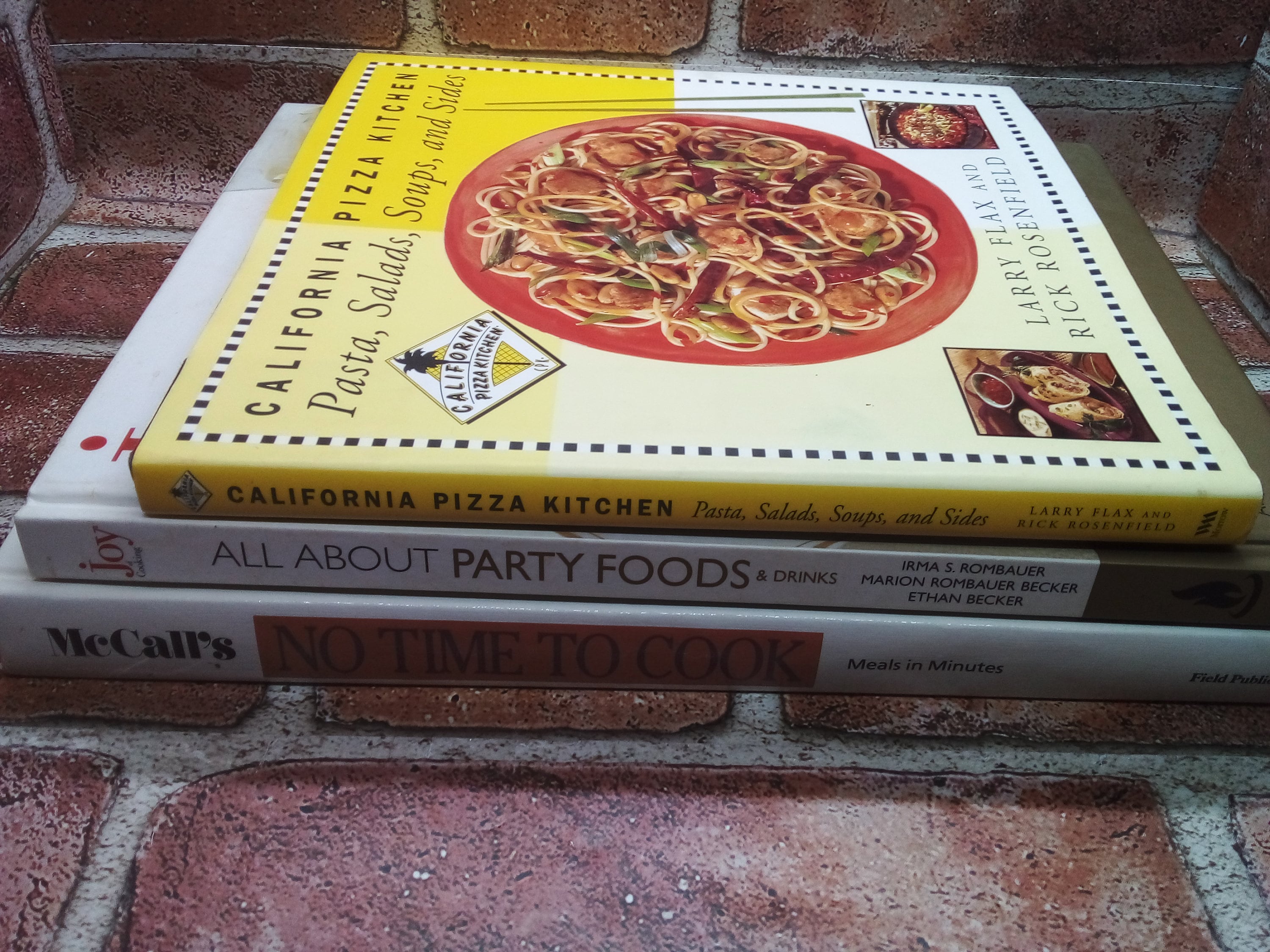This image showcases a neatly stacked trio of cookbooks positioned on a red brick slab, the grout between the bricks distinctly white. Each book in the stack diminishes in size as it advances upward. The topmost book features a vibrant yellow cover adorned with an image of a red bowl filled with spaghetti, possibly depicting a dish like shrimp scampi or chicken scampi with chili peppers. Titled "California Pizza Kitchen Pasta, Salad, Soups and Sides," it’s authored by Larry Flax and Rick Rosenfield. Beneath it lies a book with a white spine emblazoned with "All About Party Foods," part of "Joy of Cooking" by Irma S. Rombauer. The largest book at the bottom is McCall's "No Time to Cook, Meals in Minutes," identifiable by its white spine and red logo. The setting evokes a brick oven ambiance, suggesting a cozy, culinary backdrop.